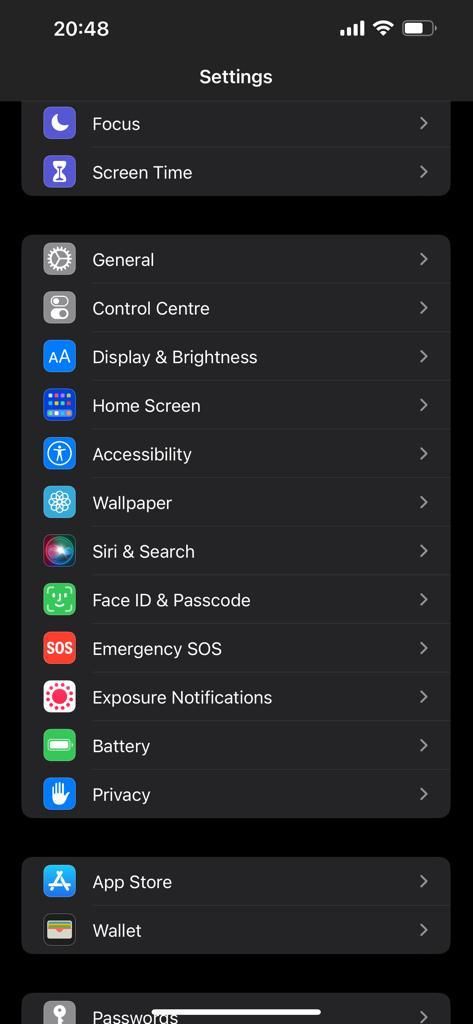In the screenshot of a mobile device displayed in this email, the time is shown as 8:48 PM at the top left corner. The top right corner features various status indicators: a fully connected network signal with 4 out of 4 bars, a strong WiFi connection with 3 out of 3 bars, and a visible battery level indicator.

The central section of the screenshot displays a settings menu encompassing several options. These options are arranged sequentially and include: 

- **Settings**
- **Focus**
- **Screen Time**
- **General**
- **Control Center**
- **Display & Brightness**
- **Home Screen**
- **Accessibility**
- **Wallpaper**
- **Siri & Search**
- **Face ID & Passcode**
- **Emergency SOS**
- **Exposure Notifications**
- **Battery**
- **Privacy**
- **App Store**
- **Wallets**
- **Passwords**

Each of these sections represents different customizable settings available on the mobile device.